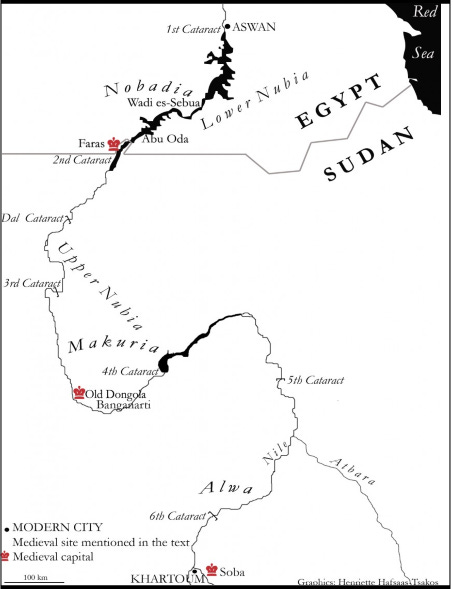This image is a detailed, hand-drawn map enclosed within a thin black frame, likely designed for a textbook or similar publication. The map depicts the geographical boundaries of Egypt and Sudan, highlighting a large wavy river which is labeled as the Nile, stretching from the top to the bottom of the image. The upper right portion of the map indicates the Red Sea, shaded in black. Various areas on the map are marked, including different towns, cities, and medieval sites.

Four small red crown symbols denote medieval capitals: one at Pharas (F-A-R-A-S) in Egypt, another at Old Dongola Banganarete, and a third one at Soba (S-O-B-A) in Sudan. The bottom of the image highlights Khartoum (K-H-A-R-T-O-U-M) as a significant landmark. Modern cities are represented as round circles, as per the legend on the map. Key locations such as Aswan and Arhamra are also labeled along the course of the Nile. This detailed map serves to illustrate both historical and contemporary geography within these regions.